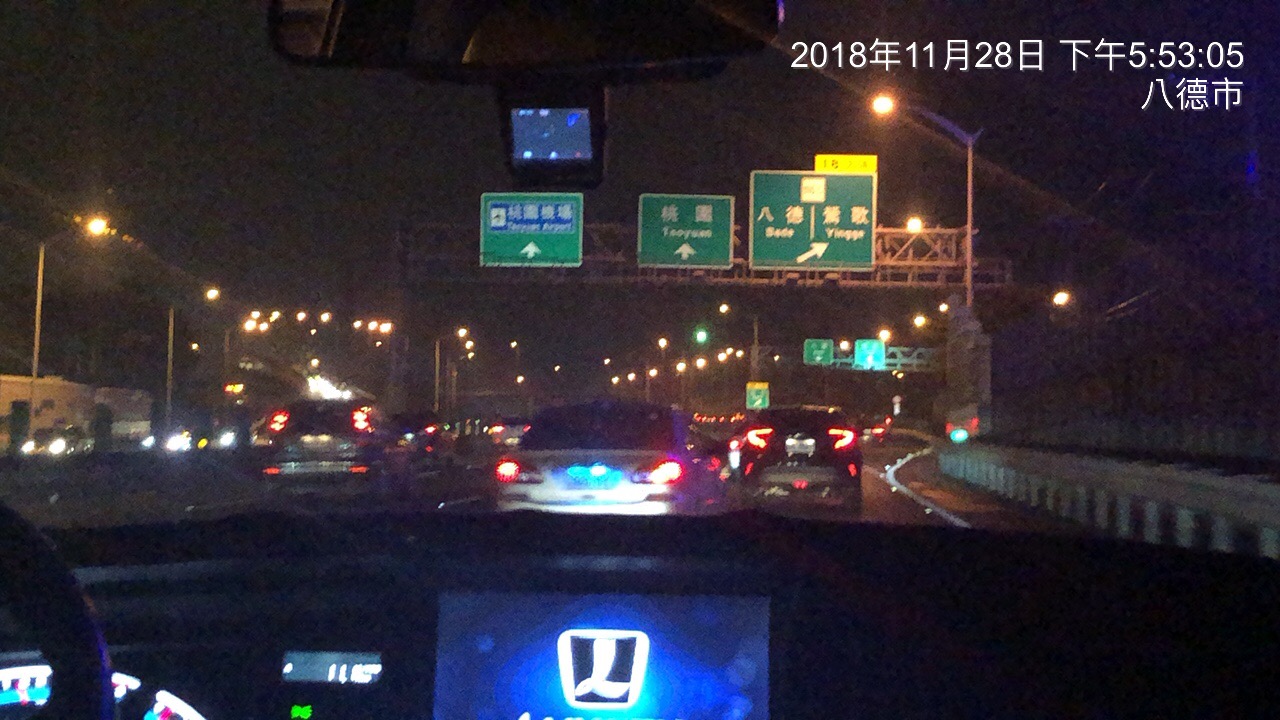This photograph captures a night scene from inside a vehicle, looking out through the windshield over the dashboard. The image displays a highway likely located in Asia, as indicated by the green and white road signs adorned with Asian characters accompanied by English translations underneath. Despite the out-of-focus nature of the photo, three distinct overhead signs can be discerned. The highway is bustling with vehicles, their brake lights glowing red against the backdrop of the darkened sky. Streetlights illuminate the road, casting a soft light over the scene. The mood conveys the essence of a lively night drive on an Asian expressway, wrapped in a blend of modern vehicular lights and traditional street signage.